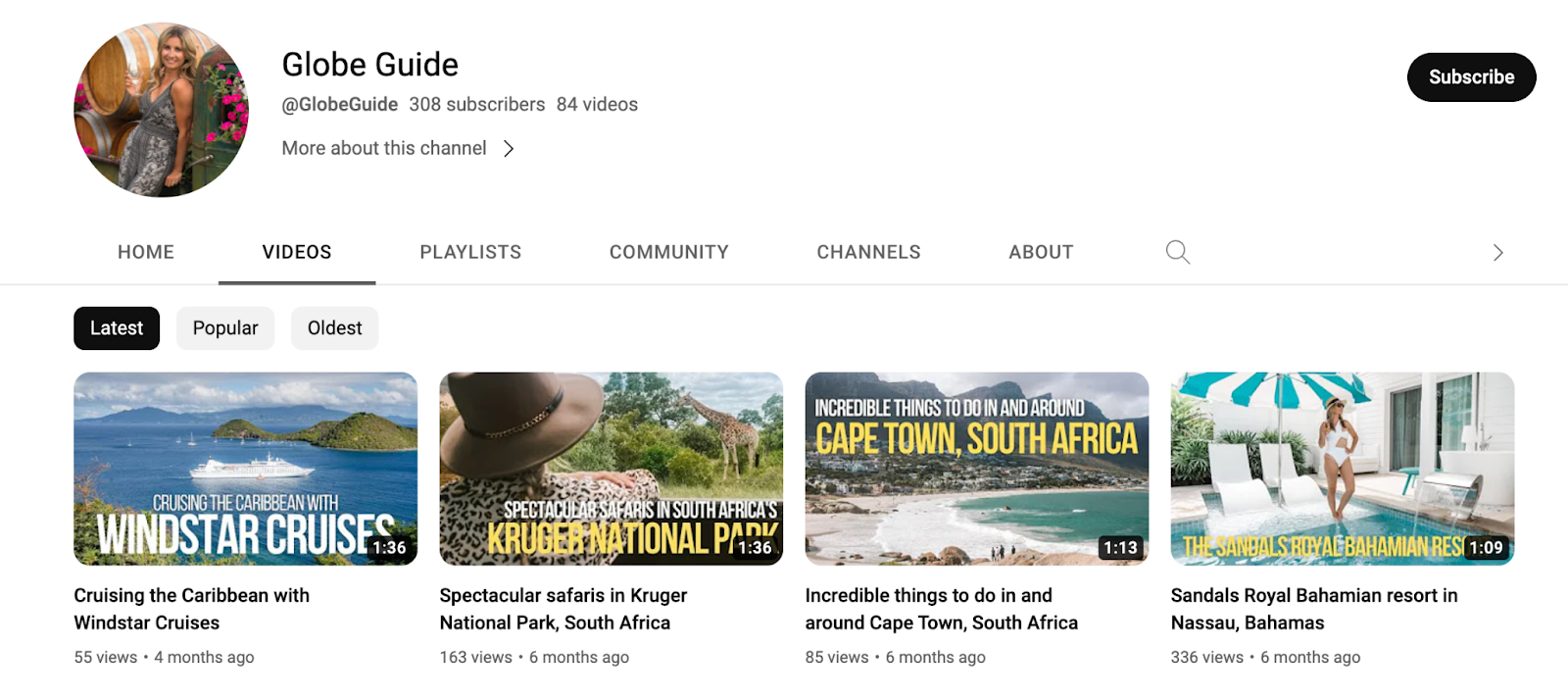Screenshot of the YouTube channel "Globe Guide" at the URL "@GlobeGuide":
- Channel Overview: 
  - Subscribers: 308
  - Videos: 84

- User Information:
  - Profile Picture: A blonde woman in a grayish-blue and white cocktail dress, seemingly photographed at a party. She is posing beside a floral bouquet featuring pink roses.

- Channel Interface:
  - Buttons Displayed: Home, Videos, Playlists, Community, Channels, About
  - Search Bar: Selected on Videos
  
- Displayed Content:
  - Viewing Mode: Desktop version, selected on Latest videos with options for Latest, Popular, and Oldest.

- Latest Video Thumbnails (left to right):
  1. "Cruising the Caribbean with Windstar Cruises":
     - Views: 55
     - Posted: 4 months ago
     
  2. "Spectacular Safaris in Kruger National Park, South Africa":
     - Views: 163
     - Posted: 6 months ago
     
  3. "Incredible Things to Do In and Around Cape Town, South Africa":
     - Views: 85
     - Posted: 6 months ago
     
  4. "Sandals Royal Bahama Resort in Nassau, Bahamas":
     - Views: 336
     - Posted: 6 months ago

- Subscriber Status: The screenshot indicates the viewer is not currently subscribed to the channel.